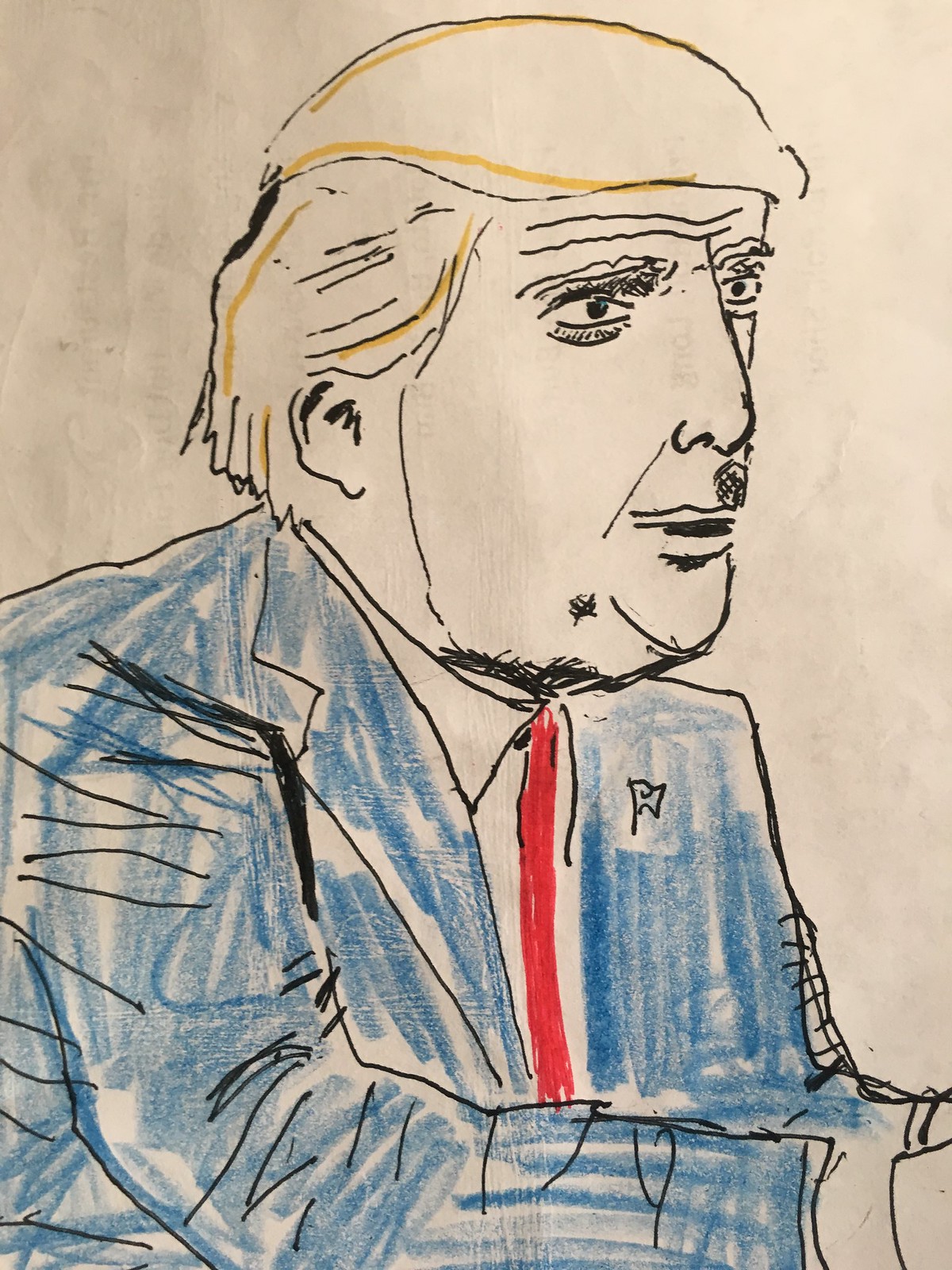This detailed drawing of Donald J. Trump appears to be a positive portrayal, though not of the highest quality. The artist has captured Trump's iconic golden lion-like hair and proportionally large head without exaggeration of his features. He is depicted wearing a blue suit and a red tie, complemented by a small American flag pin on his lapel. The coloring of the suit is done rather quickly and has an amateurish feel to it, suggesting that a younger artist might be behind this creation. Despite its simplicity, the image is fully colored and conveys a respectful nod to the former President.